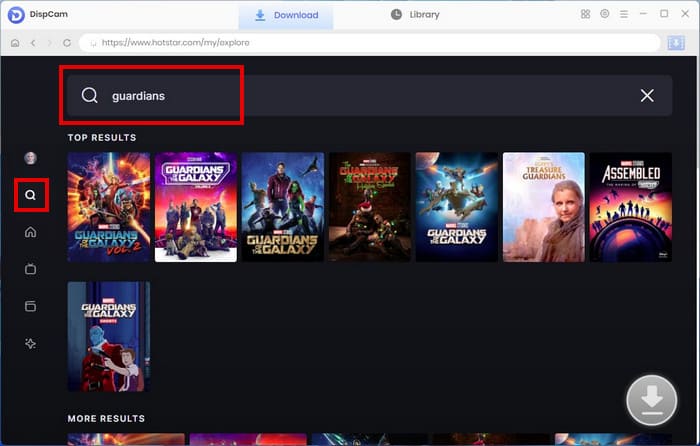This is a screenshot from the website DispCam. The top-left corner features a "D" logo encased in a blue circle. The interface includes options such as "Download" and "Library." The website's URL is https://www.hotstar.com/my/explore, displayed in the browser's address bar. Just below the top navigation, there is a search bar with the term "guardians" entered, highlighted by a red outline. The search results are prominently displayed underneath, featuring multiple thumbnails for popular media. These results include "Guardians of the Galaxy Vol. 2," "Guardians of the Galaxy Vol. 1," "Guardians of the Galaxy" in other variations, "Treasure Guardians Assembled," and an additional entry titled "Guardians of the Galaxy."